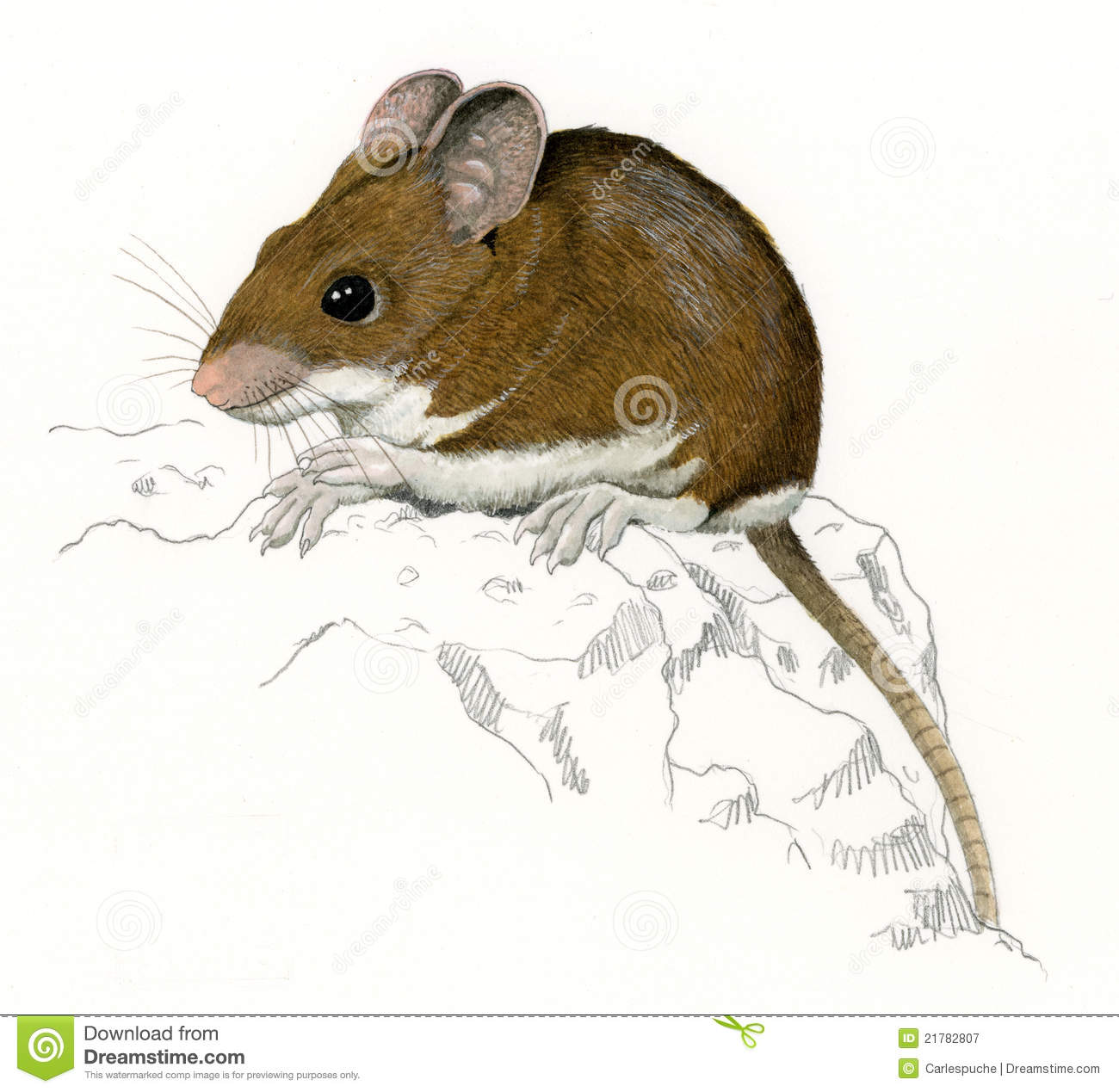This is a detailed, hand-drawn color illustration of a brown mouse, accented with subtle gray and white highlights. Its underbelly and tiny hands are white, while its ears and nose are a dull pink. The mouse's dark eyes have reflective white dots, adding a lifelike quality. It has long, thin whiskers, oval-shaped ears with gray speckling, and a long, grayish-brown tail with faint horizontal stripes that transitions to a nearly hairless tip. The mouse, perched on a black-and-white, pencil-sketched pile of rocks resembling a cliff, exudes a sense of realism despite the sketchy background. The stock image features a visible watermark from Dreamstime.com, with a perforated line indicating where the watermark would be removed upon purchase. The image ID is 21782807, and it is credited to "carlspush" and Dreamstime.com, with additional identifiers and logos along a white banner at the bottom edge.